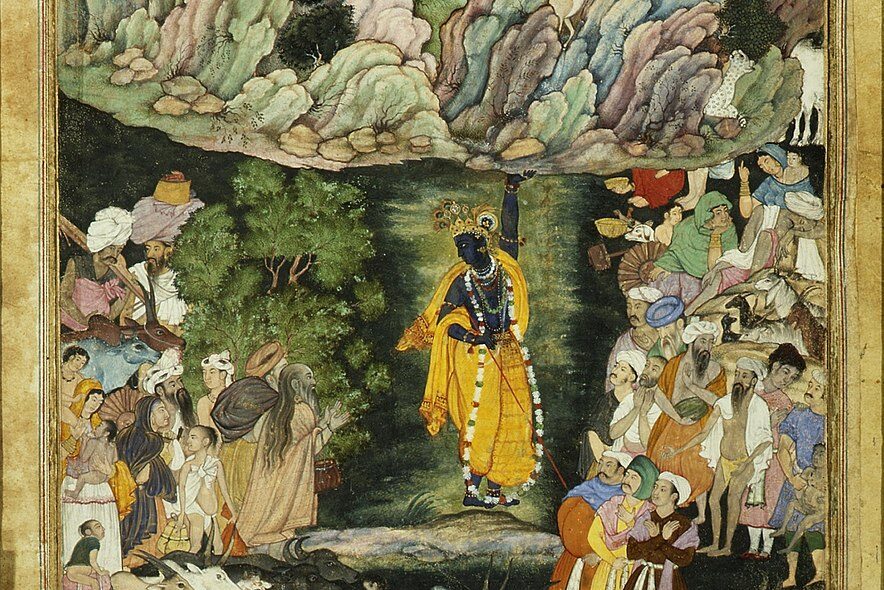This intricate Mughal-style painting, partially framed in gold on the right and left, features a striking depiction of an Indian god or deity with jet-black skin, adorned in resplendent cultural attire. At the center stands the deity, garbed in a luminous yellow robe or sari, with an ornate gold crown accented by a flowing veil and vibrant peacock feathers. The deity is heavily adorned with elaborate jewelry, including a long white beaded necklace that touches the ground, intermixed with red, green, and brown beads. The deity's bare chest is accentuated by various colorful necklaces and bracelets on the ankles.

Raising his left arm, the deity holds up a large, complex rock formation with varying hues of green, blue, brown, red, and black, alongside what appears to be trees and greenery. The background is an intense, dark greenish-black, which starkly contrasts with the deity’s vibrant outfit and the gathered crowds.

To the left and right of the deity, multiple groups of people, possibly devotees, are depicted in fine detail. These individuals have lighter skin tones and are dressed in traditional Indian attire, including turbans, headscarves, bangles, and loincloths. They are engaged in various activities, and some carry baskets or wear tall turbans. Among them, there are references to animals, including cows and donkeys, adding to the rich tapestry of the scene. The lush greenery and detailed rock formations in the background further enhance the artistry of this painting.